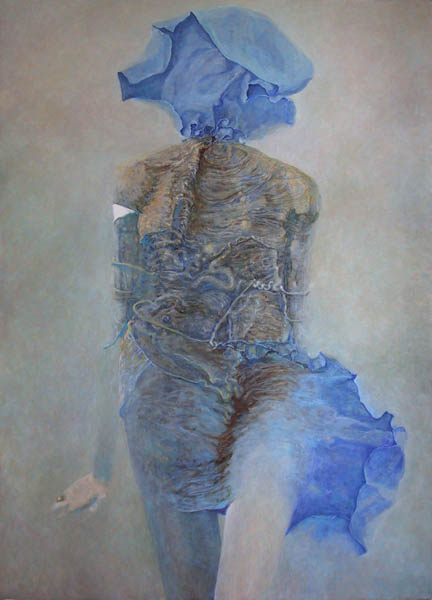A striking and enigmatic painting depicts a veiled woman with a blue fabric covering her face, rendering her features almost ghostly and disembodied. The veil is draped over her head, cascading down to obscure her face with ethereal translucence. Her attire morphs from a brownish fabric over her shoulders into various shades of blue, giving a sense of fluidity and movement as though stirred by a gentle breeze. The dress appears to dissolve into abstract shapes and serpentine forms, almost mummy-like, wrapping around her torso and down to her legs.

One of her bare legs is partially visible, stretching out from beneath the flowing blue fabric, while the other leg, enveloped in a teal hue, extends straight down. Her left hand, adorned with a ring, extends to the side in a graceful yet ambiguous gesture. Above her left elbow is a pinkish triangle cut-out, adding to the painting's unconventional texture and fragmented nature. The background transitions from reddish shadows at the top to a grayish tone towards the bottom, complementing the soft, faded, and predominantly beige and blue palette.

The painting's overall composition gives an impression of softness and decay, with intricate lines suggesting decomposition and creating an unsettling, fantastical quality. The artistic choice of nebulous patterns and colors imbues the artwork with an otherworldly beauty, leaving an indelible, enigmatic impression on the viewer.